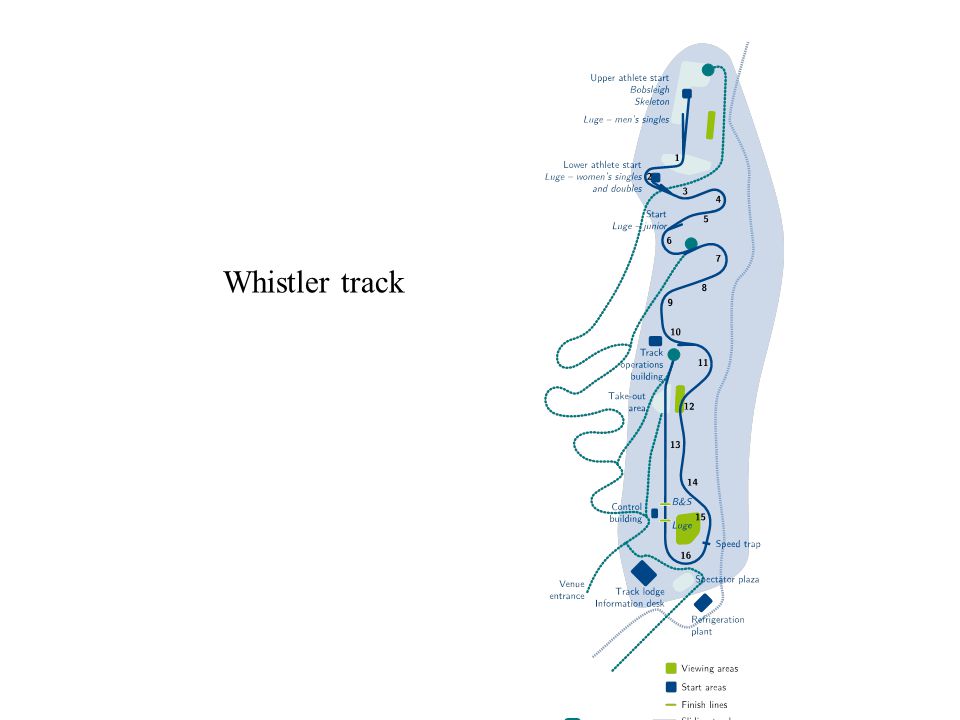This illustration depicts a vertical, oblong map of a bobsled and luge track on a light blue background. On the left side, "Whistler Track" is written in black text on a white background. The track itself is rendered as a cartoon-like image with blue lines that snake from top to bottom, representing the course's 16 numbered turns. Alongside the track, black numbers mark each turn, and specific start areas are highlighted for various events such as Bobsleigh, Skeleton, and different Luge categories. There are vibrant color-coded sections: green areas indicate viewing zones, blue squares mark start areas, and green lines signify finish lines. The map includes descriptive text labels for various operational and spectator facilities like the Track Operations Building, Spectator Plaza, and Viewing Areas. A color-coded legend at the bottom clarifies these zones, enhancing the map's detailed and informative layout.